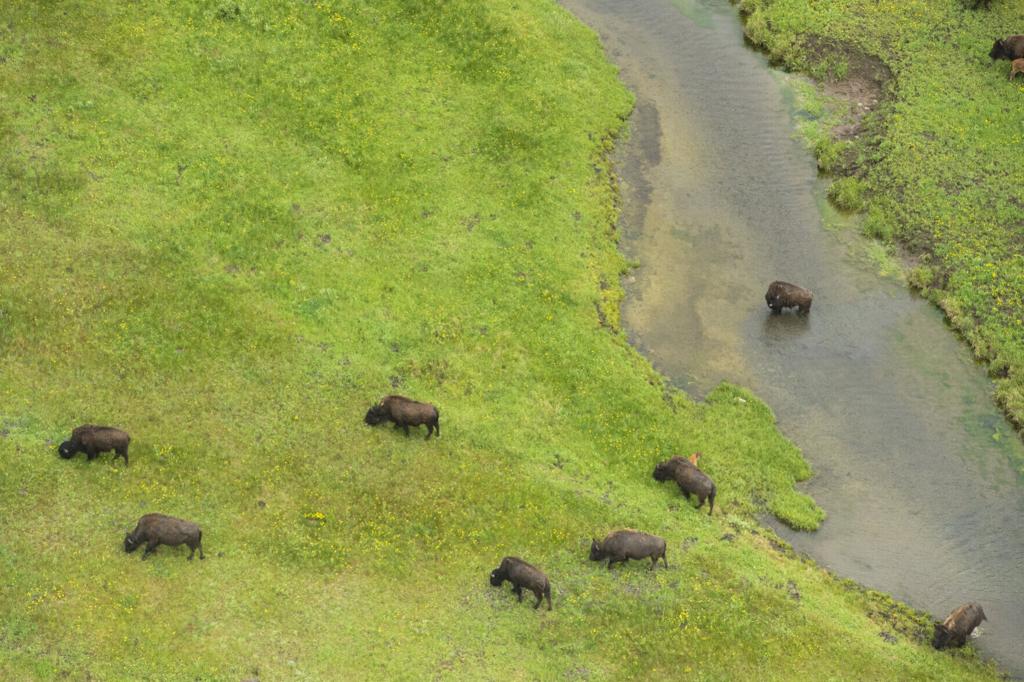This is a color aerial photograph capturing a bird's-eye view of a serene, natural tableau featuring eight buffalo, possibly water buffalo. They are scattered across a verdant landscape, with a river flowing on the right side of the image. The river's banks are lush with grass, exhibiting varying shades of green and patches of yellow, possibly from blooming flowers.

One buffalo is positioned in the middle of the river, gazing towards the others, while another is in the process of crawling out of the water at the very lower right-hand corner of the frame. The remaining six buffalo are dispersed across the grassy land, leisurely grazing. This tranquil scene combines elements of nature and wildlife, with the buffalo immersed in their pastoral routine amidst the rich, green terrain.